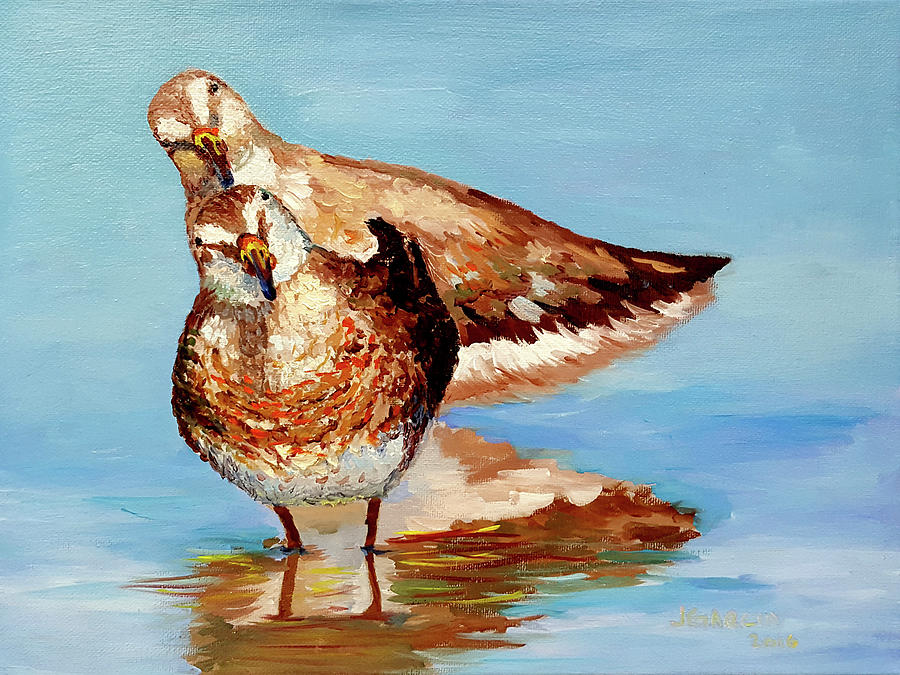This detailed oil on canvas painting features two ducks, or possibly birds of a similar kind, serenely situated on a wavy blue water surface. The focal point of the artwork captures both birds standing close together, with delicate reflections beneath them, adding a sense of depth to the image. One duck is positioned in the foreground looking straight ahead, while the other stands slightly behind, turned perpendicularly to the left but with its head also directed straight ahead. 

Their heads are cocked to the right, giving them a curious and attentive appearance. The coloration of the ducks is meticulously rendered: their faces are white with dark brown heads and necks. Their wings exhibit a mosaic of beige, light brown, and reddish hues, transitioning into darker brown at the tips. The birds' bellies are primarily white with faint brown spots leading to their vivid orange-yellow beaks. 

The background sky, painted in a light blue with and white, seamlessly blends into the reflective water below, enhancing the overall serene atmosphere of the painting. The artist’s signature, located at the bottom right corner, is somewhat indistinct but seems to read "J-G-A-R-E-R" with a possible date of either 2006 or 2016.